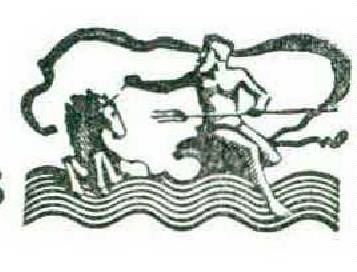The image appears to be an intricate black and white or grayscale drawing that evokes ancient or mythological themes. Dominating the right side of the composition is a figure resembling Poseidon or Neptune, identifiable by his trident held in his left hand. He is depicted nude and seated, possibly on a rock or a wave element that seamlessly blends into the flowing water beneath him, indicated by seven distinct wavy lines.

The mythological figure reaches with his right hand towards a unicorn positioned slightly to his left. Both man and beast engage in a mutual gaze, creating a striking focal point. The unicorn is lying down, with subtle horn details that affirm its identity as a mythical creature. 

This dynamic interaction is enveloped by swirling lines and shapes that emanate from Poseidon/Neptune, enveloping the unicorn and adding a sense of motion and fluidity to the scene. The artwork is rendered in simple, yet evocative, lines and shadings, suggesting the use of monochromatic ink or pencil, devoid of any additional colors, enhancing its timeless and classic appearance.